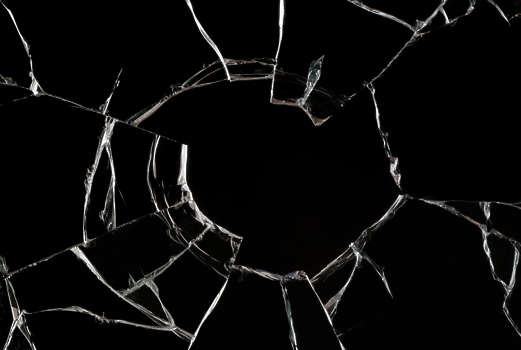This detailed photograph depicts a close-up view of a broken pane of clear, colorless glass set against a completely solid black background. The glass has a significant, roughly baseball-sized hole at its center, suggesting it was shattered by an object—perhaps a ball or a rock—thrown through it. Radiating outward from the central hole, numerous cracks and fractures extend to the edges of the glass, creating an intricate, web-like pattern reminiscent of a spider web. Some of these fractures are intersected by additional lines, enhancing the chaotic yet mesmerizing look of the shattered glass. The stark contrast between the dark background and the gleaming white reflections along the cracks highlights the details of the breakage, emphasizing the dramatic impact and intricate shattering pattern.